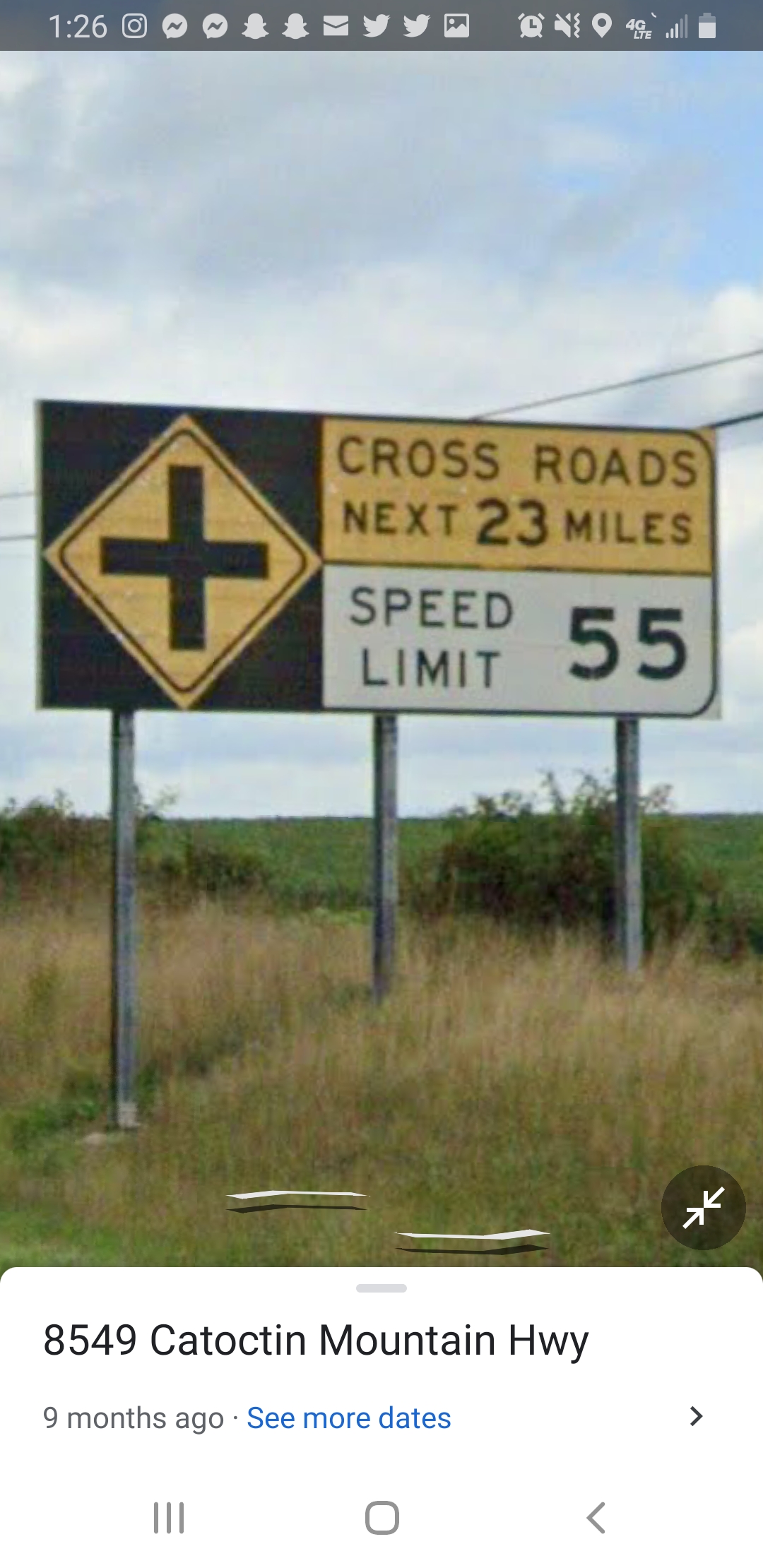The image captures a screenshot of someone's phone screen, timestamped at 1:26, with a multitude of icons at the top such as Twitter, an envelope, notifications, and various others. Displayed on the phone is a country setting photograph taken midday under a partially cloudy sky with some blue peeking through. The landscape shows a mix of green and tan grasses in what looks like a meadow, with a few white objects scattered in the foreground and trees or bushes in the distant background.

The main focal point of the image is a highway sign supported by three gray metal posts. The sign features a yellow diamond-shaped symbol with a black intersection cross on the left. On the right side, in large black capital letters on a yellow background, it reads "CROSS ROADS NEXT 23 MILES." Below this, in a white section, the text states "SPEED LIMIT 55." At the bottom of the sign is another white section displaying "8549 Catacoctin Mountain Highway" with the note "nine months ago" and an option to "see more dates," printed in blue.